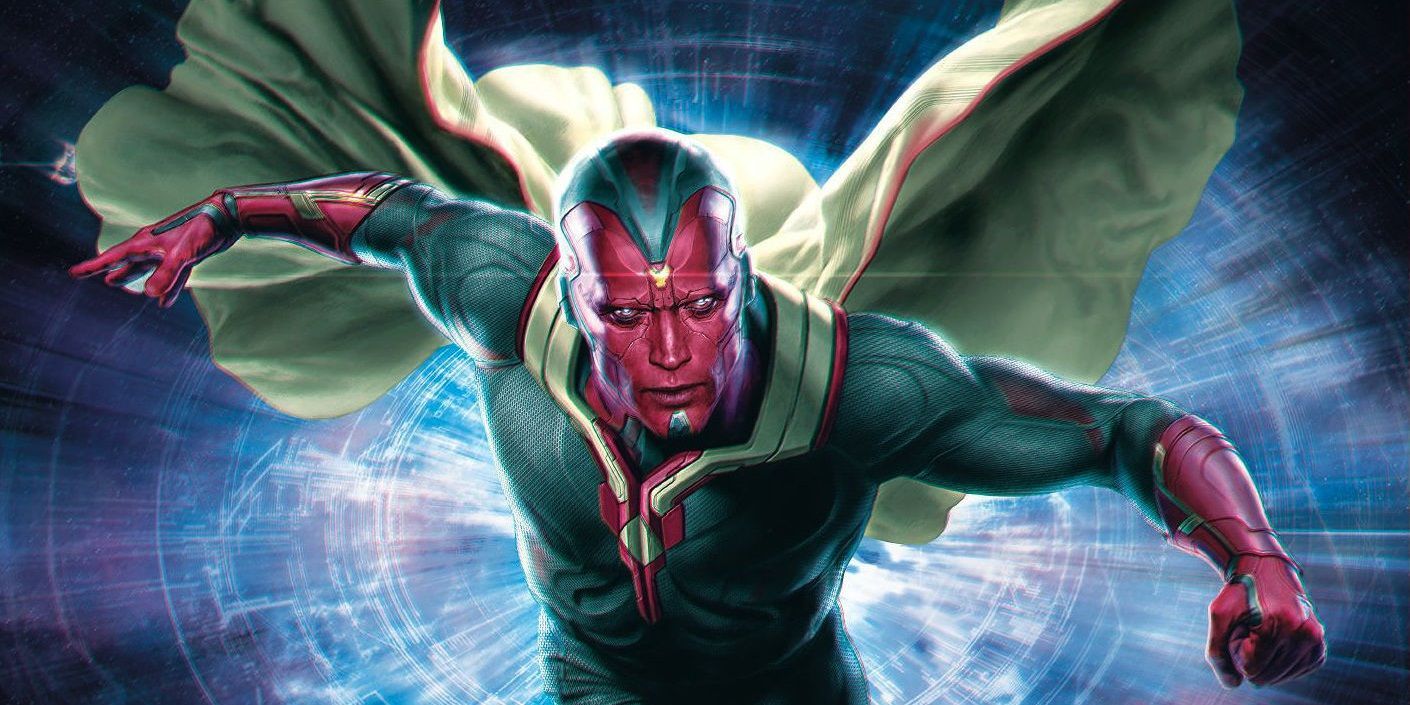In this vibrant 3D-rendered image, a digitally created superhero takes center stage with a striking combination of red and green elements. The character sports a green form-fitting suit complemented by a dynamic, flowing green cape edged with red hues. His face is predominantly red, with yellow eyes and a distinct yellow icon centered on his forehead just above the long nose. His head is topped with a green helmet, and his strong, red-clad arms are raised, one hand clenched into a fist, evoking a sense of power and readiness.

The superhero's red gloves and slightly green-tinted chin, resembling a goatee, add to his detailed and colorful appearance. He stands boldly against a dramatic background marked by an explosion-like burst of white light, radiating in concentric circles and straight lines, creating a vivid contrast against the predominantly black surroundings. This animated, cartoon-style image is text-free and captures the essence of a character that is a fascinating blend of attributes reminiscent of both Superman and Green Lantern, set outdoors with an intense and glowing backdrop.